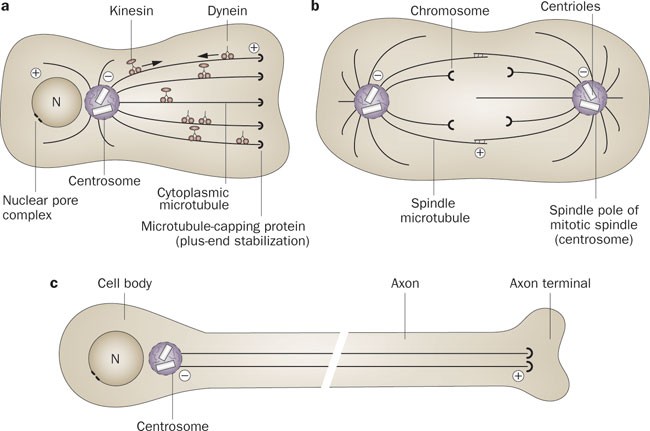This illustration, seemingly from a biology textbook, presents three detailed diagrams labeled A, B, and C, portraying different cellular structures with labels identifying various components. 

In image A, the focus is on intracellular components including the centrosome, nuclear pore complex, kinesin, dynein, and cytoplasmic microtubules, illustrating the intricate machinery of cellular operation. Picture B highlights the elements involved in cell division such as the chromosome, centriole, spindle pole, meiotic spindle, and spindle microtubules, showcasing the dynamic organization during the mitotic process. Image C depicts a neural cellular structure, emphasizing the cell body, centrosome, axon, and axon terminal, which are crucial for nerve signal transmission. 

The entire illustration employs muted, subdued colors, predominantly tans, purples, and whites, giving it a scientific and procedural appearance that aligns with its educational purpose.